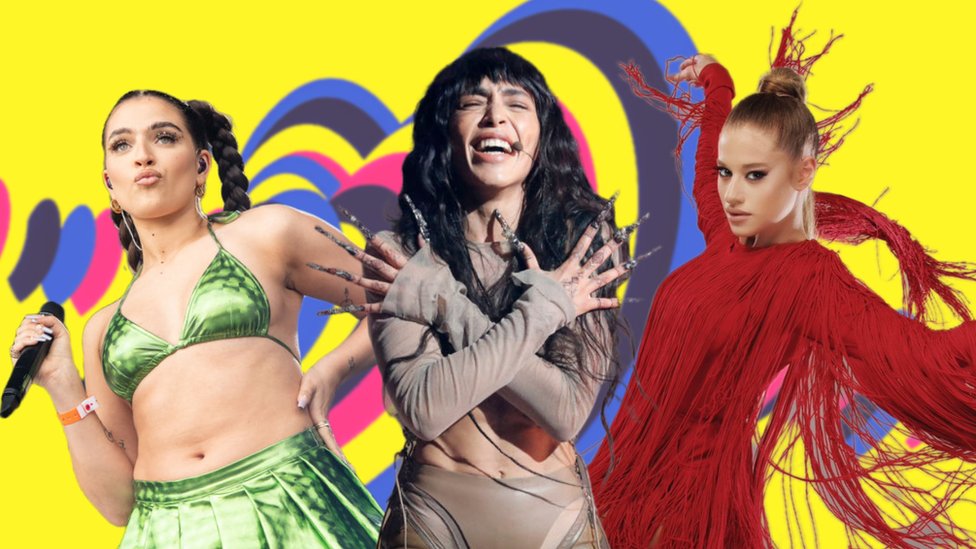The image depicts a visually striking promotional photograph featuring three women, likely musicians, set against a vibrant yellow background adorned with dark blue, light blue, pink, and purple heart-like abstract patterns. The women appear to have been individually photographed and later composited together, as they do not seem to be standing naturally next to each other.

The woman on the left is Caucasian, wearing a shiny, satin green bralette and a pleated skirt. She has braided pigtail plaits, an orange wristband on her right hand, and holds a microphone, suggesting she's a singer. Additionally, she has a hearing device in her left ear.

In the center stands the second woman, possibly the winner of Eurovision 2023 from Sweden, dressed in a beige bodycon outfit that reveals her midriff. She is adorned with extremely long, colorful nails, likely six inches in length, giving a dramatic flair to her appearance. She has very long black hair with waves and bangs, and is wearing a headphone set that indicates she’s performing on stage.

On the right is a young Latina woman clad in a flamboyant red dress with intricate fringe details, resembling a flamenco-style outfit. Her hair is styled in a top knot, and she poses gracefully with her arms raised like a ballerina.

The combination of these elements, along with their individual dynamic poses, suggests a cohesive yet artistically composite image intended to promote a musical event or group performance, possibly linked to Eurovision.